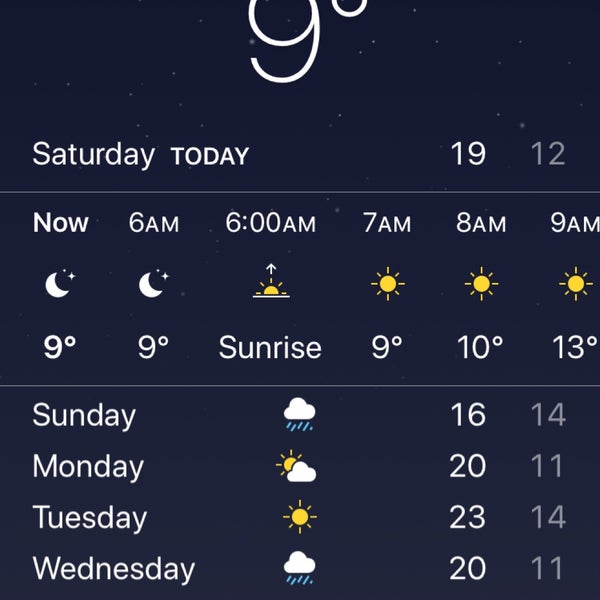A detailed weather application interface is displayed against a dark gradient background of deep black and blue hues resembling a night sky, adorned with tiny star-like specks. Dominating the top center of the screen is the large, bold number "9," representing the current temperature of 9 degrees. Directly beneath this, the day is specified as "Saturday," along with the forecasted high and low temperatures - 19 and 12 degrees respectively.

Further down the screen, the app provides an hourly forecast starting with the current temperature of 9 degrees. The following hours are listed as 6 a.m., 7 a.m., 8 a.m., and 9 a.m., along with their corresponding temperatures of 6, 7, 8, and 9 a.m. showing 9, 10, and 13 degrees respectively. Each hour also features an icon displaying a bright sun, indicating clear, sunny weather for the morning hours.

At the bottom of the display, a four-day forecast is presented for Sunday, Monday, Tuesday, and Wednesday. Sunday is depicted with a cloud and raindrops, suggesting rain showers, while Monday shows a cloud partially covering the sun, indicating partly cloudy weather. The forecast includes the high and low temperatures for each of these upcoming days, providing a comprehensive overview of the weather for the next few days.